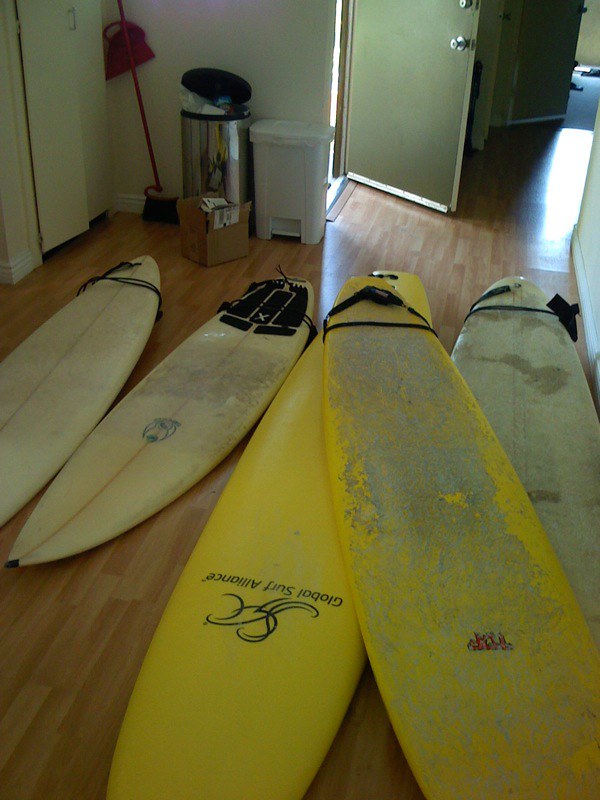This color photograph depicts the interior of a room with five surfboards laid out on a light brown, striated wooden floor. The image is slightly underexposed, enhancing the sunlight that streams in from an open green door, creating highlights on the floor towards the top right portion of the image. 

In the background, against the wall, sits an overfilled trash can accompanied by another white rectangular trash bin. Nearby, a leaning lamp with a brown shade and a standing broom emphasize the domestic setting. The surfboards themselves, showing signs of wear with grainy textures and scratches, are likely being prepared for sale.

Two shorter white boards with brown center stripes and black footings lie to the left; the board on the far left is partially cut off. One of these has a visible blue logo. To the right, two much longer yellow boards are positioned, one emblazoned with "Global Surf Alliance" on its top surface, while the other, likely showing its more scratched underside, features no distinctive markings. Atop these, another white board, similar in appearance to the first, lies at an angle. Each board's unique characteristics and conditions are prominently displayed on the wooden floor of this lived-in space.